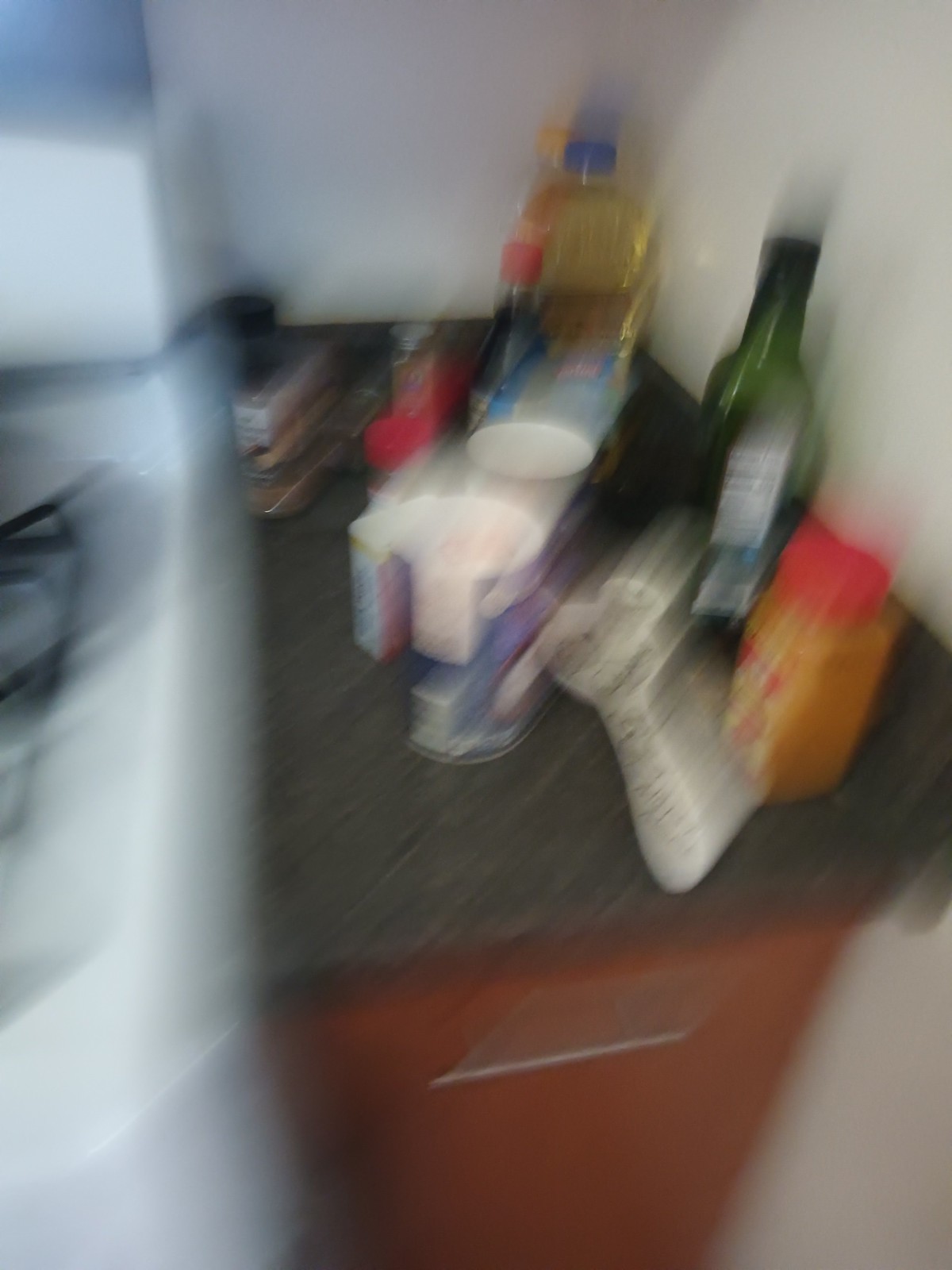The image is an extremely blurry photograph of a kitchen counter, giving the impression that the camera moved significantly as the photo was taken. On the left side of the image, a white stovetop oven with black grating is partially visible. Adjacent to the stove is a slim kitchen counter, composed of a gray countertop and medium warm brown shelving beneath it. The counter holds a variety of kitchen items, including a plastic jug of canola oil, a green bottle of olive oil, a large spice mix, a mixing spoon, and several tubs, though some items are too indistinct to identify clearly. The wall behind the counter is plain white. To the left of the scene, there might be a window, lending some ambiguity to the setting. Additionally, there's mention of a long, horizontally placed brass-colored handle on a drawer, as well as vague forms resembling cylindrical and rectangular containers that could be for seasonings like salt and pepper. An electrical cord may also be present in the scene, contributing to the cluttered array of cooking-related goods.